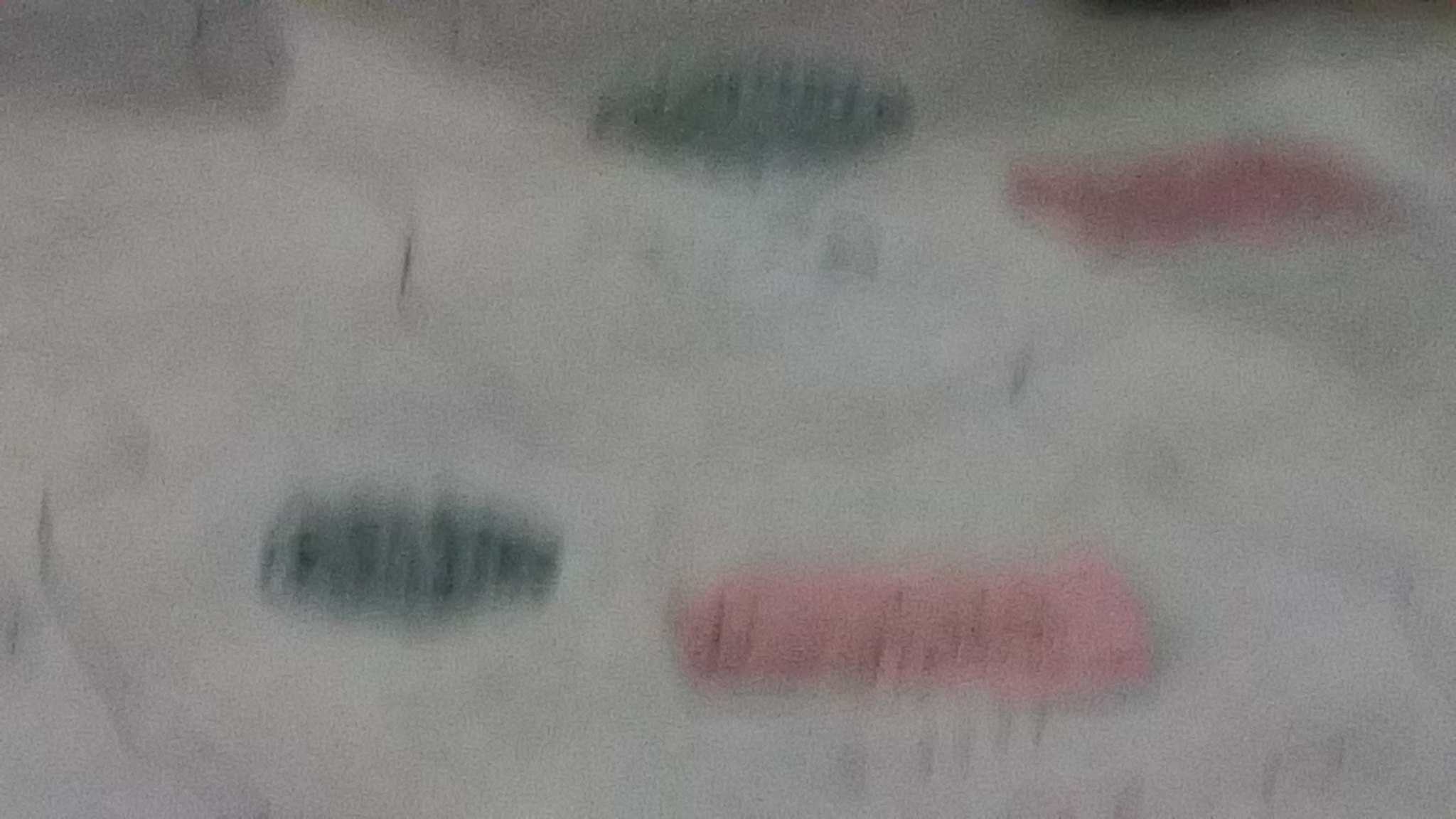This extremely blurry and grainy image features several indistinct shapes on a predominantly white background. There are rectangular pink pieces of paper scattered across the top right and bottom right of the photo, laying on what appears to be either a table or white fabric. Two horizontally elongated green ovals are also present, with one positioned at the top center and the other towards the left of the frame. The lower left quadrant features a round green blur, while the upper center has another similar green shape. Black smear lines can be seen towards the left side of the image, and there is a noticeable shadow in the top right corner, contributing to the overall sense of visual noise and distortion.